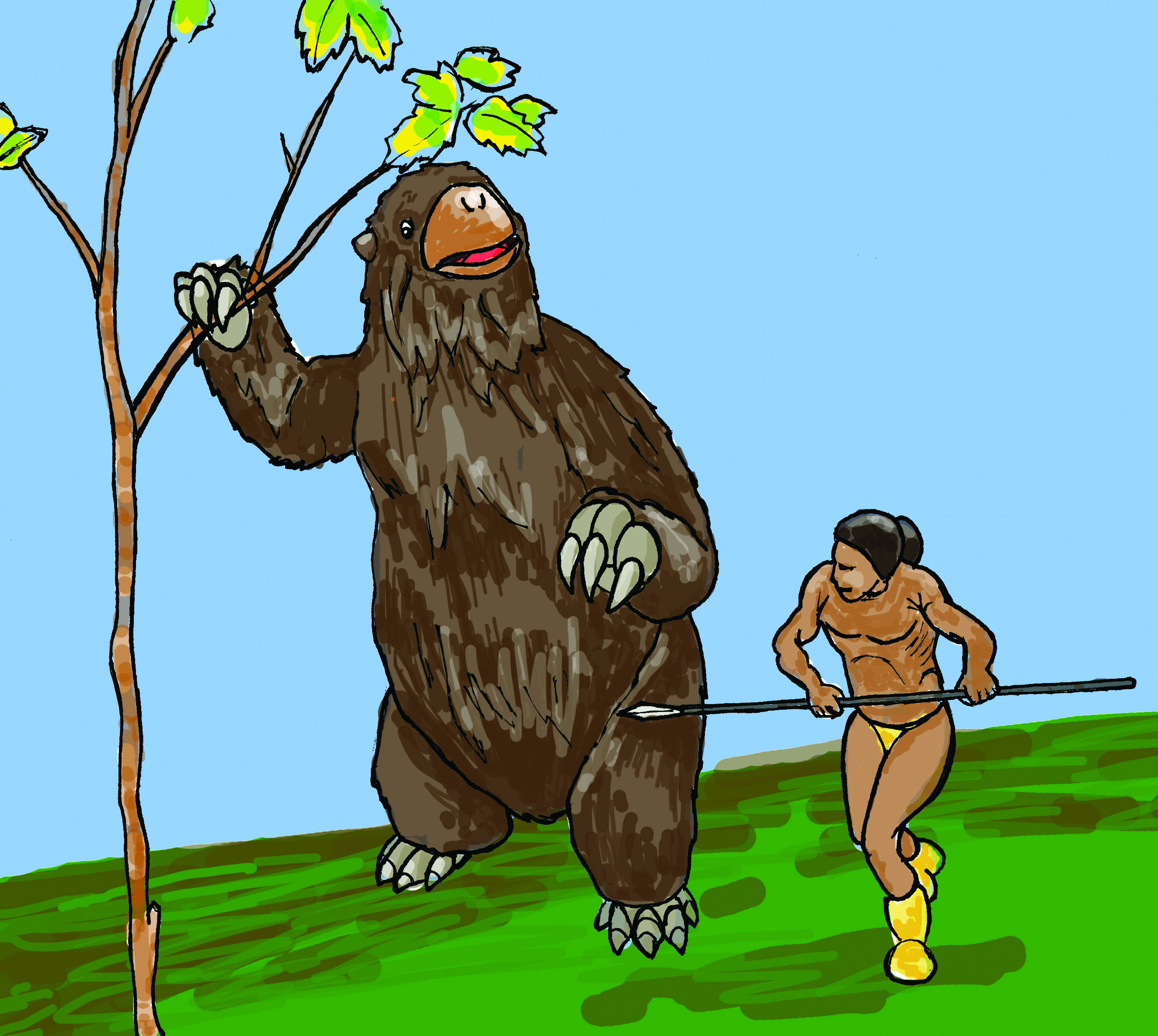The illustration is a crude drawing depicting a dramatic scene in a green landscape with a blue sky. At the center of the composition, a large, brown, furry creature, resembling a giant sloth with black eyes, a brown nose, and three significant claws on each paw, clings to a slim tree with its right arm, looking distressed. Opposite this creature, a human figure, whose gender is ambiguous, charges with a spear in both hands. This individual has a medium skin tone, long black hair tied back, and is minimally clothed, wearing only a yellow loincloth and yellow boot-like footwear. The human appears to be attacking the giant sloth, whose mouth is open, revealing a red tongue, as if in a moment of fear or surprise.